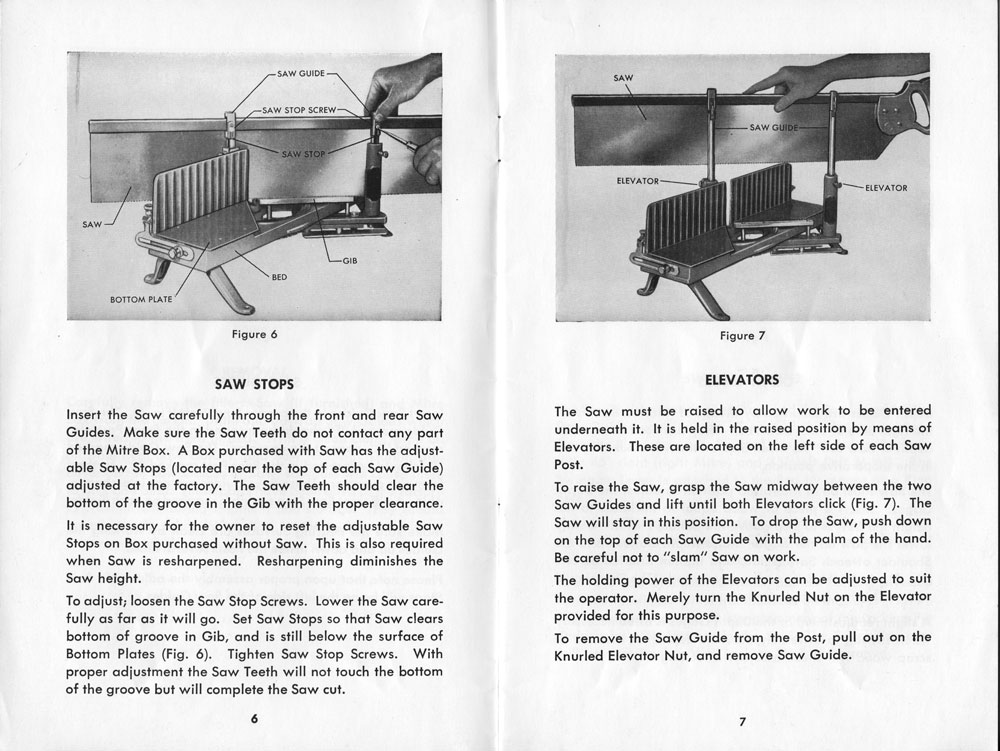This is a detailed photograph of two pages from an old, black and white manual, featuring comprehensive instructions on using a SawStop and a SawElevator. Both pages are topped with diagrams; the left page is titled "Saw Stops," and the right is labeled "Elevators." Each diagram shows a piece of equipment being handled and labeled with parts such as the saw guide, SawStop screw, and bottom plate.

The left page depicts a man's hand holding a screwdriver and adjusting the SawStop screw. The accompanying text provides detailed instructions on the correct use of the SawStop. It explains how to insert a saw through the front and rear saw guides without allowing the teeth to touch any part of the mitre box, and it includes safety guidelines and adjustment procedures.

On the right page, another diagram shows a saw held by a man's hand, illustrating the use and components of the SawElevator, marked with labels like elevator and saw guide. The text beneath elaborates on the process of raising the saw to begin work, ensuring safe operation.

Each page is supplemented with three or more paragraphs of instructional text, making it a rich, informative guide for users of these tools.